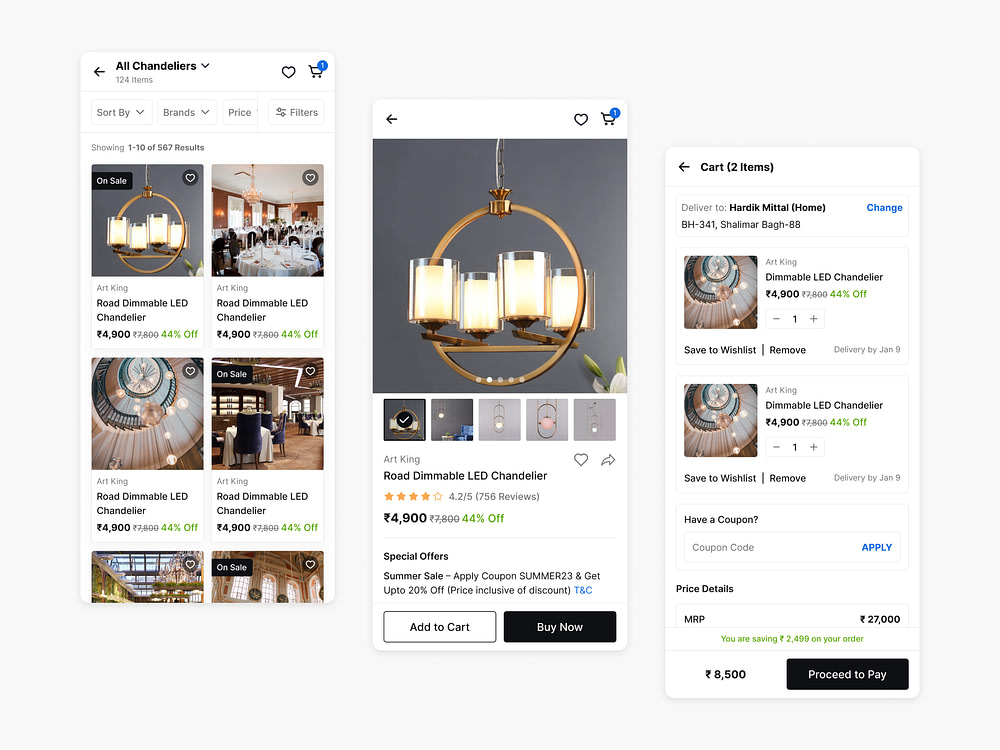The image comprises three screenshots from a shopping app, focusing on chandeliers. The leftmost screenshot displays an assortment of chandelier options under the category "All Chandeliers." Each chandelier is accompanied by a thumbnail image, showcasing various styles and designs. The central screenshot zooms in on a specific chandelier that the user has selected. This chandelier is identified as a "Road Dimmable LED Chandelier," with a price tag of 4900 units in an unspecified currency, accompanied by a section labeled "Special Offers" that likely highlights any ongoing promotions or discounts. The rightmost screenshot reveals the user's shopping cart, which contains two different chandeliers, providing a summary view of the items chosen for potential purchase.